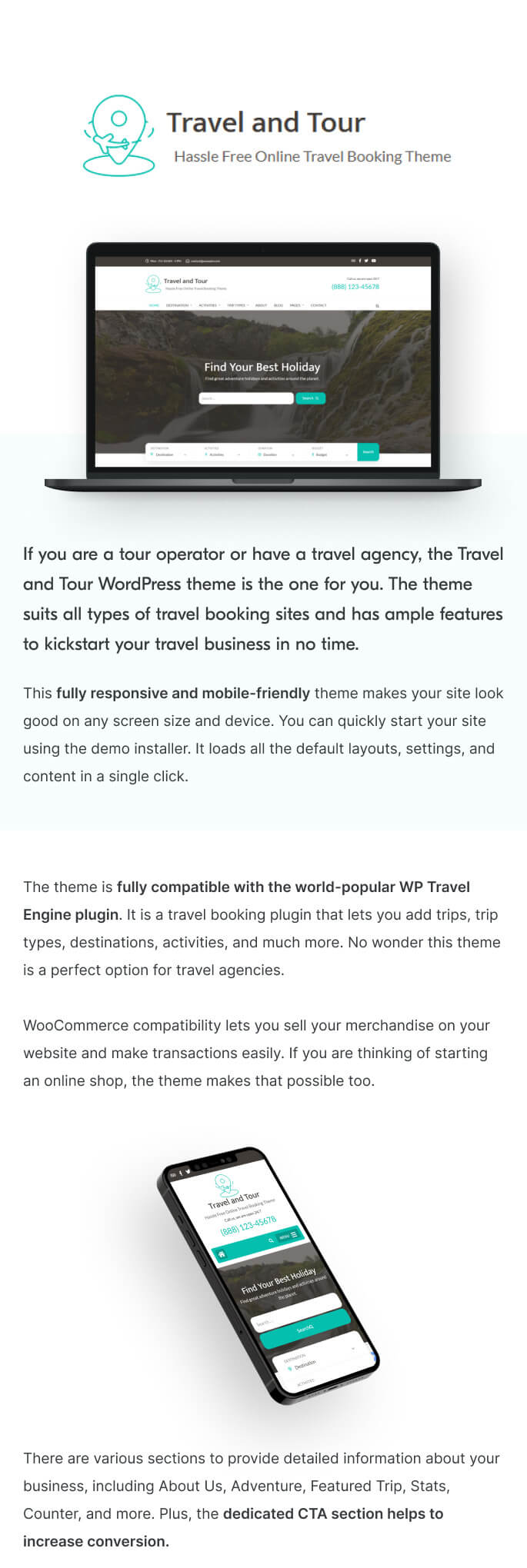This webpage features a centered header that reads "Travel and Tour," followed by a tagline below it stating "Hassle-free Online Travel Booking Theme." The main visual element is an image of a laptop, also centered, displaying the text "Find Your Best Holiday" along with a white search bar. Below the laptop image, there is a description aimed at tour operators and travel agencies, highlighting the Travel and Tour WordPress theme. This theme is designed for various types of travel booking sites and boasts numerous features to help you kick-start your travel business swiftly.

Further down, the description emphasizes that this fully responsive and mobile-friendly theme ensures your site looks great on any screen size and device. It mentions the convenience of using the demo installer to quickly set up your site with default layouts, settings, and content with a single click. Additionally, the theme is fully compatible with the widely-used WP Travel Engine plugin. This plugin enables you to add trips, trip types, destinations, activities, and much more, making it an ideal choice for travel agencies looking to enhance their online presence.

Overall, the Travel and Tour WordPress theme provides a robust and user-friendly solution for anyone in the travel industry, from tour operators to travel agencies, to create an attractive and functional travel booking site.